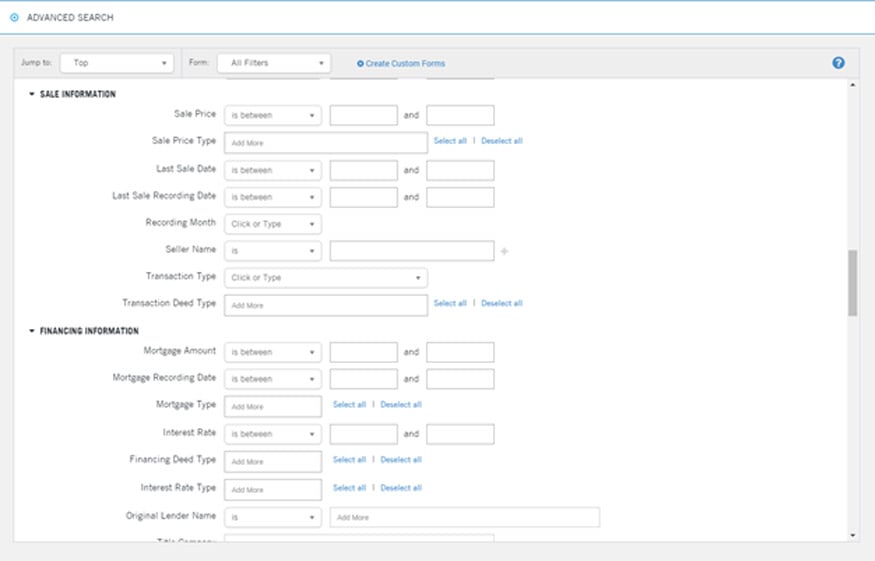The image depicts a colorful, yet functional website interface, designed for advanced search capabilities. The layout is straightforward, prioritizing usability over style. Positioned at the top left, the text "Advanced Search" indicates the purpose of the page: allowing users to perform detailed searches based on specific criteria.

Users can navigate the page via a "Jump to" feature, which currently highlights the "Top" option, potentially signifying navigation preferences like top, bottom, or center of the page. Users can select "All filters," enabling a comprehensive search, with the additional option to create custom forms tailored to individual needs.

The interface is divided into two main sections: "Sale Information" and "Financing Information."

### Sale Information:
- **Sale Price**: Users can specify a range (e.g., between X and Y).
- **Sale Price Type**: Options can be selected categorically.
- **Last Sale Date**: Input the most recent sale date.
- **Last Sale Recording Date**: Record the last date of sale documentation.
- **Recording Month**: Choose the month the recording took place.
- **Seller Name**: Information about the seller's identity.
- **Transaction Type**: Classify the nature of the transaction.
- **Transaction Deed Type**: Type of deed involved in the sale.

### Financing Information:
- **Mortgage Amount**: Specify a range or exact amount.
- **Mortgage Reporting Date**: Date when the mortgage was reported.
- **Recording Date**: The date the mortgage was officially recorded.
- **Mortgage Type**: Type of mortgage (e.g., fixed, variable).
- **Interest Rate**: Specify the interest rate.
- **Interest Rate Type**: Whether the rate is fixed, variable, etc.
- **Financing Deed Type**: Type of financing deed used.
- **Original Lender Name**: The name of the original lending institution.

These features collectively ensure users have the tools and options needed for precise searches relevant to sales and financing specifics.